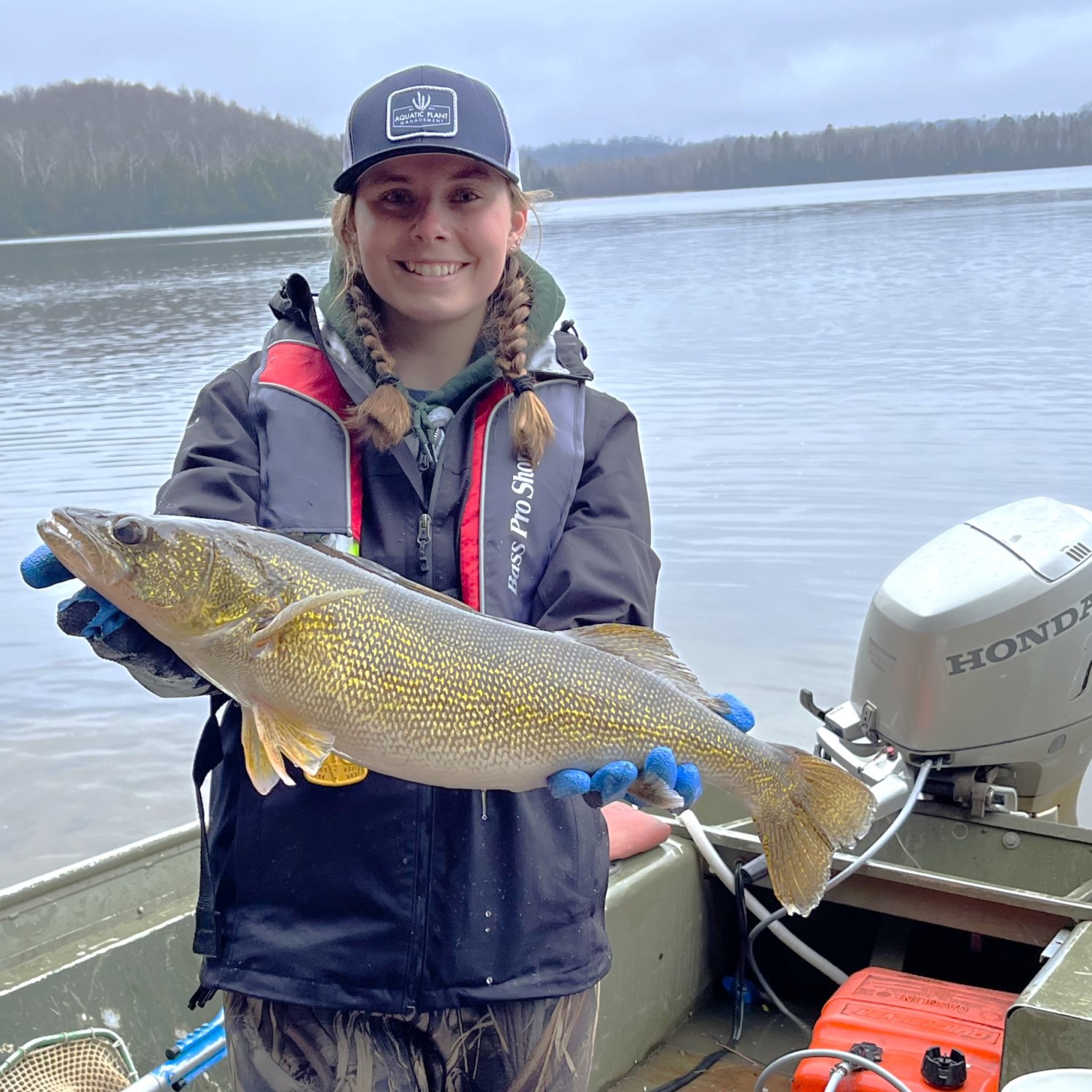In this vibrant daytime photograph, a young woman stands triumphantly in a small fishing boat on a serene lake, framed by a backdrop of hills with fall foliage and bright blue skies. She is outfitted in a navy blue Bass Pro Shop weatherproof jacket with red accents and a matching navy blue baseball cap. Her blonde hair is styled in pigtails, and she is beaming proudly as she displays her impressive catch – a stunning gold and brown fish, estimated to be about 24 to 30 inches long with shimmery scales. The fish is held securely in her royal blue-gloved hands, its head in her right hand and its tail in her left. The boat, equipped with a Honda outboard motor, contains a red gas canister, a fishing net with a blue handle, and some unidentified orange object. The calm blue waters of the lake and the partially bare, green-tinted trees in the background suggest an early fall setting.